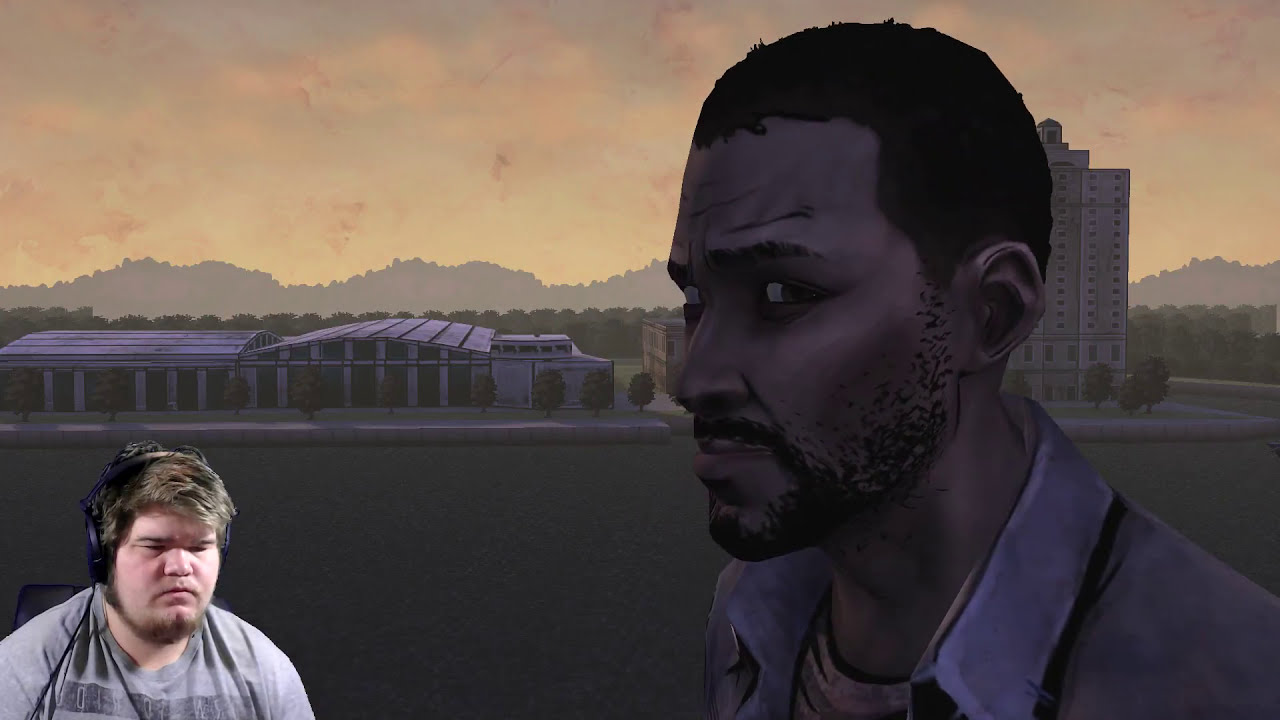In this detailed video game screenshot, we see a scene from the game "The Walking Dead," featuring the main character, Lee. Lee, an African American man with short dark hair and a goatee, is looking to the right, dressed in a blue jacket over a gray shirt. The game boasts a distinctive cel-shaded, comic book art style. In the background, there are buildings and a street, framed by a field of trees leading to mountains in the distance under a mostly yellow, evening sky. 

On the bottom left of the screen, a live streamer is superimposed, indicating this scene is part of a live Let's Play session. The streamer, a young man in his 20s with a slightly heavyset build, has short brown hair and a connected full beard. He is wearing a gray shirt and black headphones while seated in a black chair, visibly engaged in the game. This setup confirms the image as a screen grab from a live stream, enhancing the immersive experience of watching and playing video games.